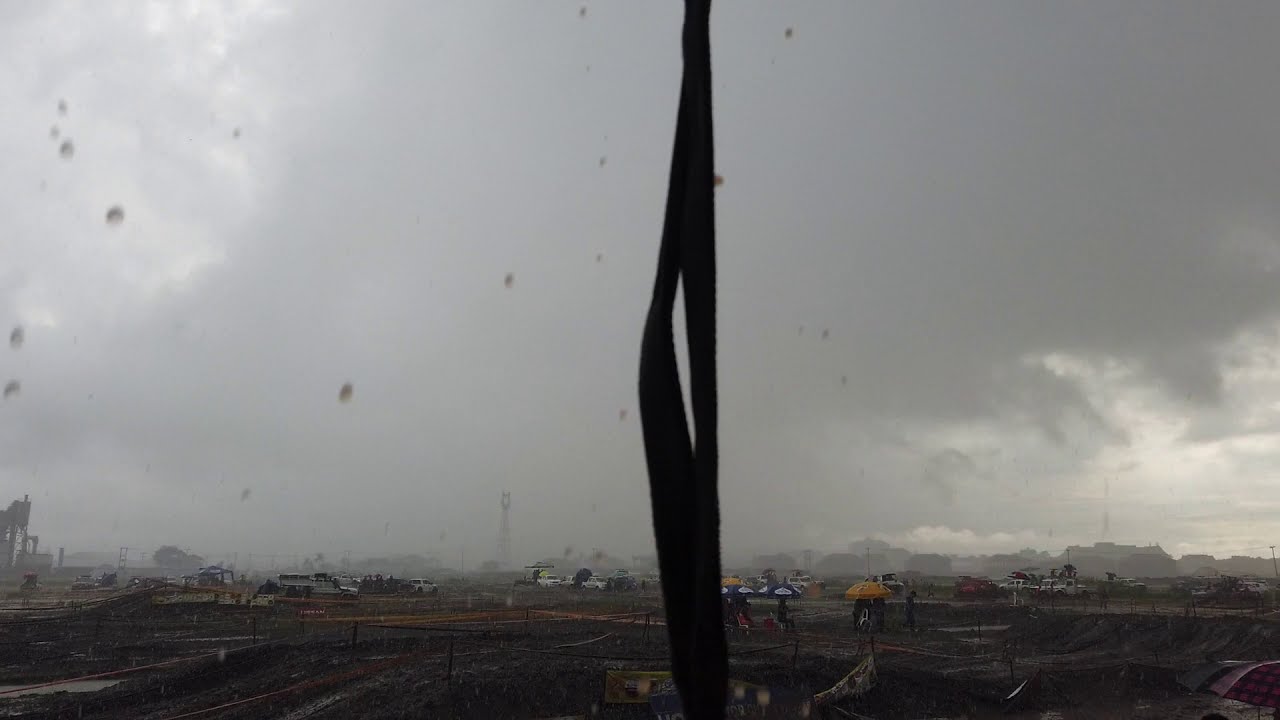The image depicts a heavily overcast, rainy day as seen from inside a car through the windshield. Raindrops are visible on the glass, especially on the left-hand side. Dominating the scene is a stormy gray sky filled with thick, heavy clouds, creating a sense of gloom. The camera captures a parking lot with wet, brown ground, where several vehicles are parked. People can be seen standing under umbrellas or canopies, adding to the dreary atmosphere. A black vertical bar, likely a windshield wiper, runs from top to bottom in the center of the image, partially obstructing the view. The background is further obscured by fog, making it difficult to make out the gray buildings and possible agricultural or factory area in the distance. The scene is devoid of any text, emphasizing the bleakness of the rainy day.